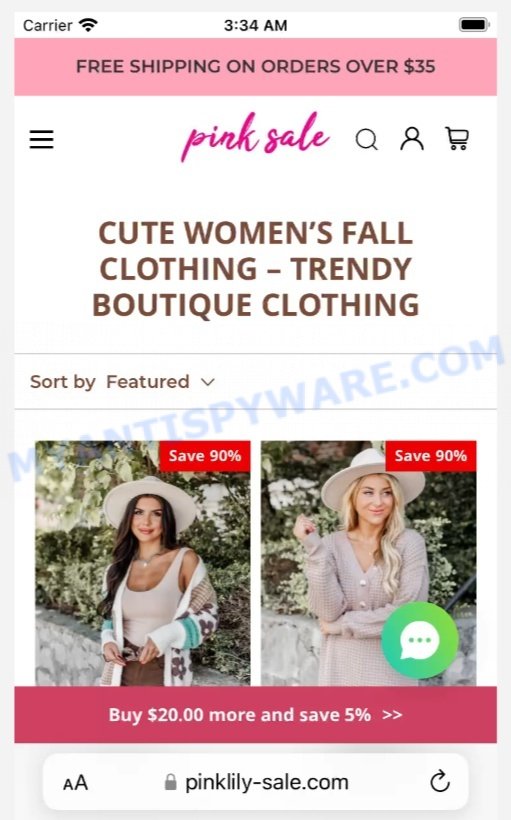A visitor navigates to a women's fashion website, evident by the detailed layout on the screen. At the top left, the current time reads 3:34, accompanied by the word "Carrier." On the top right, a battery icon appears. Beneath this header, a prominent pink banner with black text boldly announces "FREE SHIPPING ON ORDERS OVER $35," followed by a cursive text stating "Pink Sale." To the right of the banner, icons for search, user login, and a shopping cart are visible. To the left, a menu icon featuring double or triple lines is available, appearing in a brown hue.

The website's main content presents two central deals: both offer a "SAVE 90%" discount, although the exact items on sale aren't specified. The first promotional image showcases a Latina woman with long hair, adorned in a stylish white hat, a tank top paired with a floral long-sleeve shirt. Below her image, a pink banner with white text promotes an additional offer: "BUY $20 MORE AND SAVE 5%."

At the bottom of the page, contrary to typical website layouts, the site’s name "pinklilysale.com" is displayed. Next to it, another image featuring a blonde woman also advertises a "SAVE 90%" deal. A green chat button is present, indicating the availability of customer service assistance. 

Overall, the website emphasizes trendy, cute women's fall clothing and offers various sorting and searching functionalities to enhance the shopping experience.